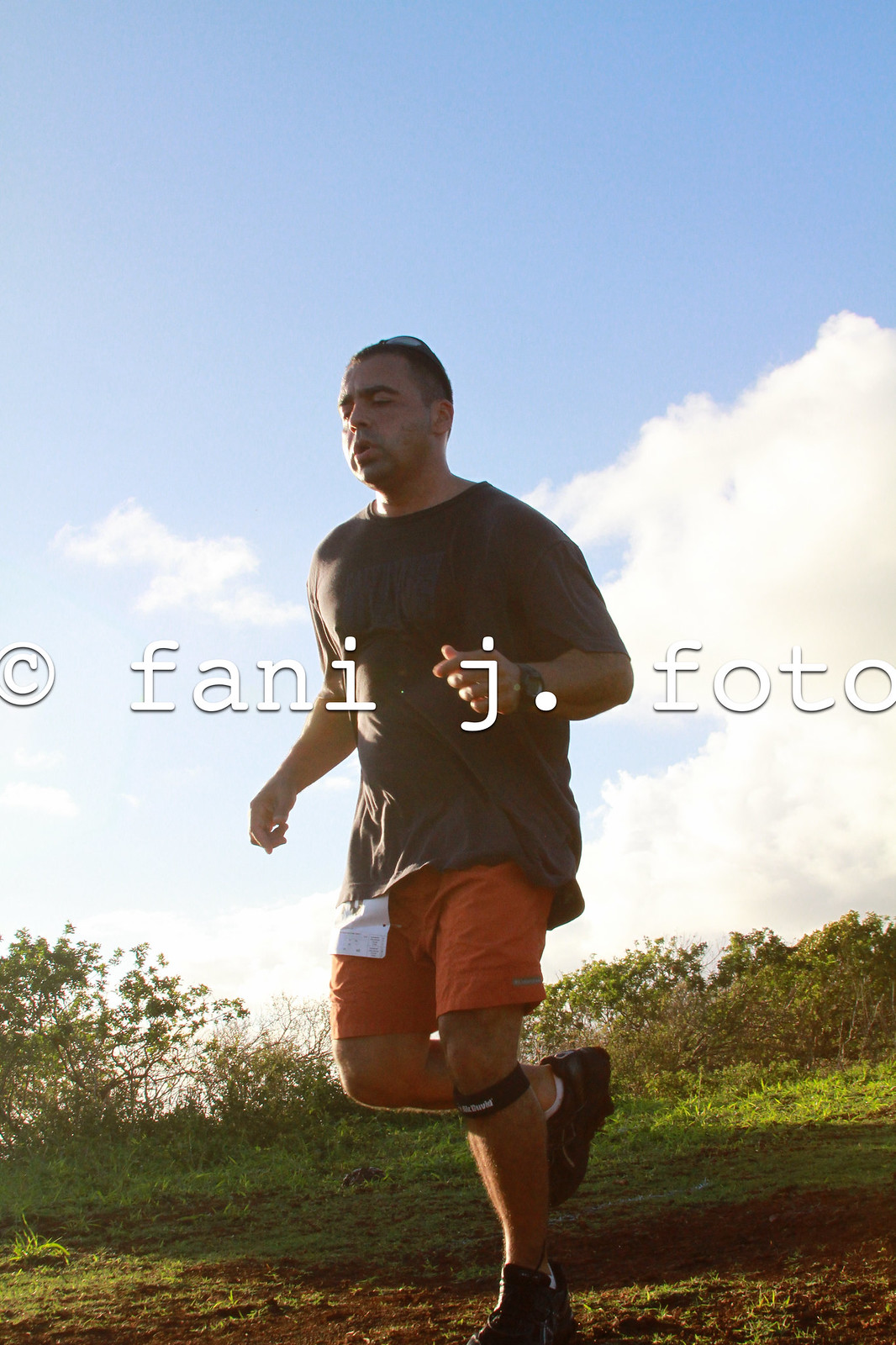In this detailed image, we see a middle-aged man in the midst of running along a brown path that transitions into green grass. His attire consists of a long dark gray t-shirt and vibrant orange shorts, with a piece of paper seemingly attached where a pocket might be. He sports black running shoes and a black band around one knee. His right leg is firmly planted on the ground while his left leg is bent, hanging in mid-air, capturing the essence of motion. The man has short brown hair with sunglasses pushed up onto his head and wears a watch on his wrist. His eyes are closed, conveying a sense of exertion. The backdrop features a clear light blue sky with a large white cloud and green weeds, trees, and bushes in the distance, adding depth to the scenery. Overlaid in white text across the center of the image is a copyright symbol, followed by "F-A-N-I J. F-O-T-O."